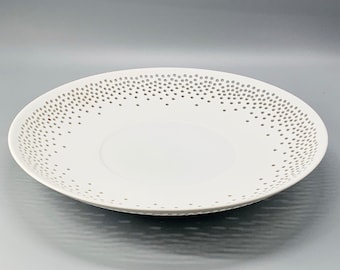This close-up photograph features an elegant white ceramic dinner plate with a slight curve, resembling a shallow bowl, on a simple gray table or flat surface. The plate is adorned with delicate gold polka dots around its edge, which gradually become sparser towards the center, leaving the middle of the plate completely white. The reflective gray surface beneath the plate creates the illusion of ripples, enhancing the visual interest of the otherwise minimalist background. Additionally, there is a shadow cast by the plate on the right side, adding depth and a secondary pattern beneath. The dots at the edge of the plate cluster closely together and disperse as they move inward, seamlessly fading into the pristine white center.